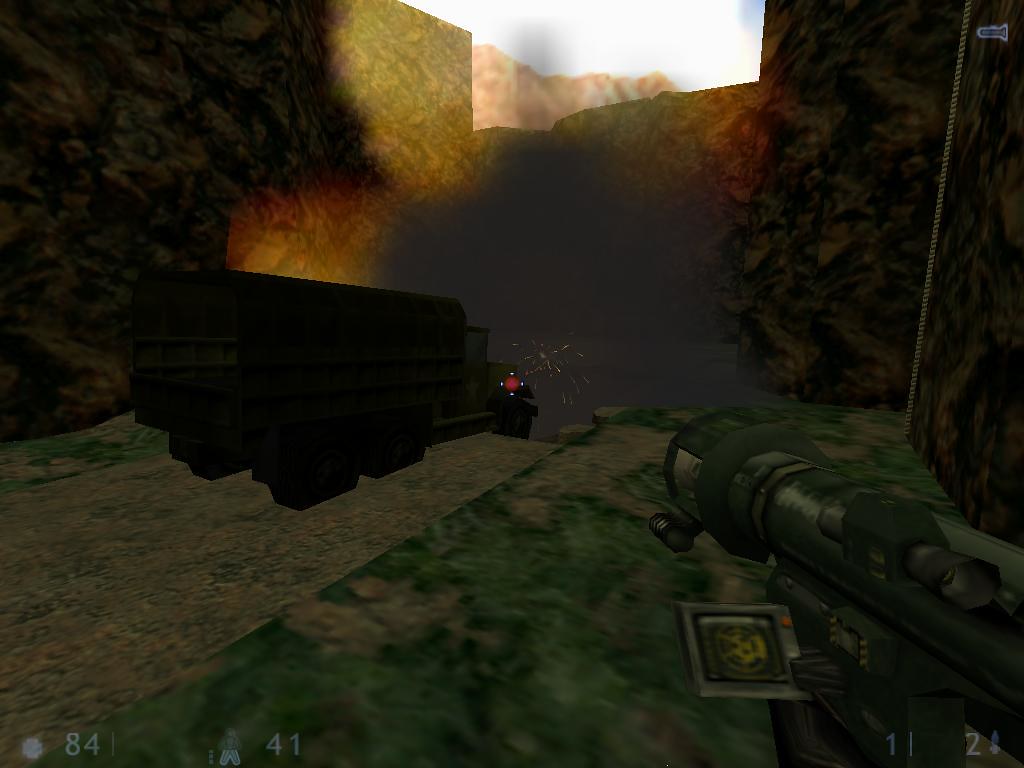In this early 2000s war-themed video game, a player character is depicted holding a bazooka, having just launched a rocket towards a truck in the distance. The truck appears to have been either hit or abandoned, as suggested by the crosshairs focused on its front and the smoke billowing out from within and around it. The environment features green patches representing grass, possibly placing the scene within a jungle. Surrounding the area are pixelated mountains or dense shrubberies, characteristic of the game's graphical style from that era.